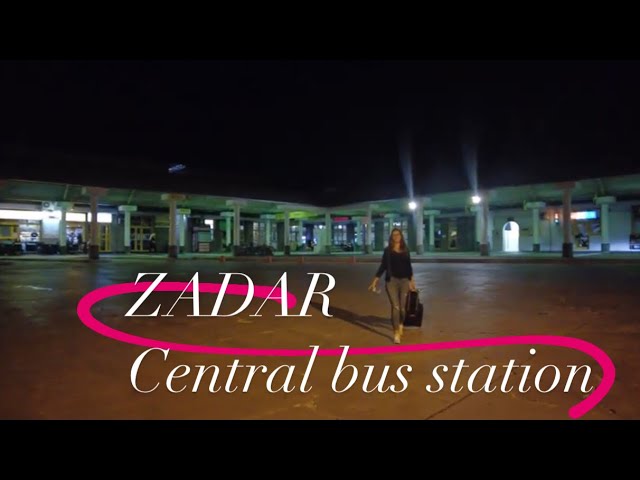In front of the Zadar Central Bus Station, a woman with shoulder-length dark brown hair is walking across a smooth, brown pavement. She is dressed in a black shirt and faded blue jeans, paired with white shoes. Her right hand clutches a black bag, while her left hand is relaxed by her hip. Above her, two bright white lights shine forward, illuminating the area against a pitch-black night sky. The station's signage in white lettering, with a distinctive curved pink line behind it, stands out prominently. In the background, the large L-shaped building features open bays for buses, supported by columns, and several lit doorways and windows can be seen. The shiny surface underfoot suggests the pavement might be wet.